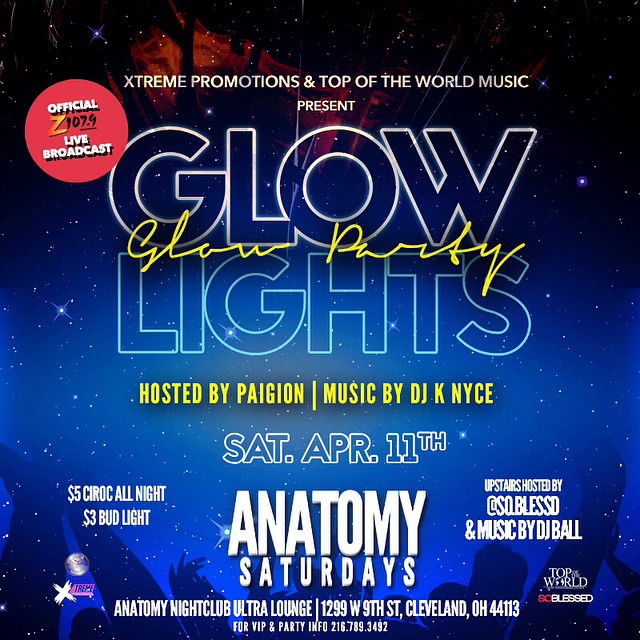Here is a cleaned-up and detailed caption, using the shared and repeated details from each person's description:

This is a promotional poster for an event titled "Glow Lights, Glow Party," presented by Extreme Promotions and Top of the World Music. The event is hosted by Paigion, with music by DJ K Nice and an official live broadcast by Z 107.9. The party is scheduled for Saturday, April 11th, at Anatomy Nightclub Ultra Lounge, 1299 West 9th Street, Cleveland, Ohio 44113, as part of Anatomy Saturdays. The poster features a striking background depicting a night sky with stars, creating an energetic and welcoming atmosphere. At the bottom, there are silhouettes of people raising their hands, simulating a lively dance party. Prominent offers include $5 Ciroc all night and $3 Bud Light. Additionally, the upstairs will be hosted by @So.Blessed with music by DJ Ball. For VIP and party information, the contact number is 216-789-3492. This poster effectively combines vivid imagery and essential event details to attract partygoers.